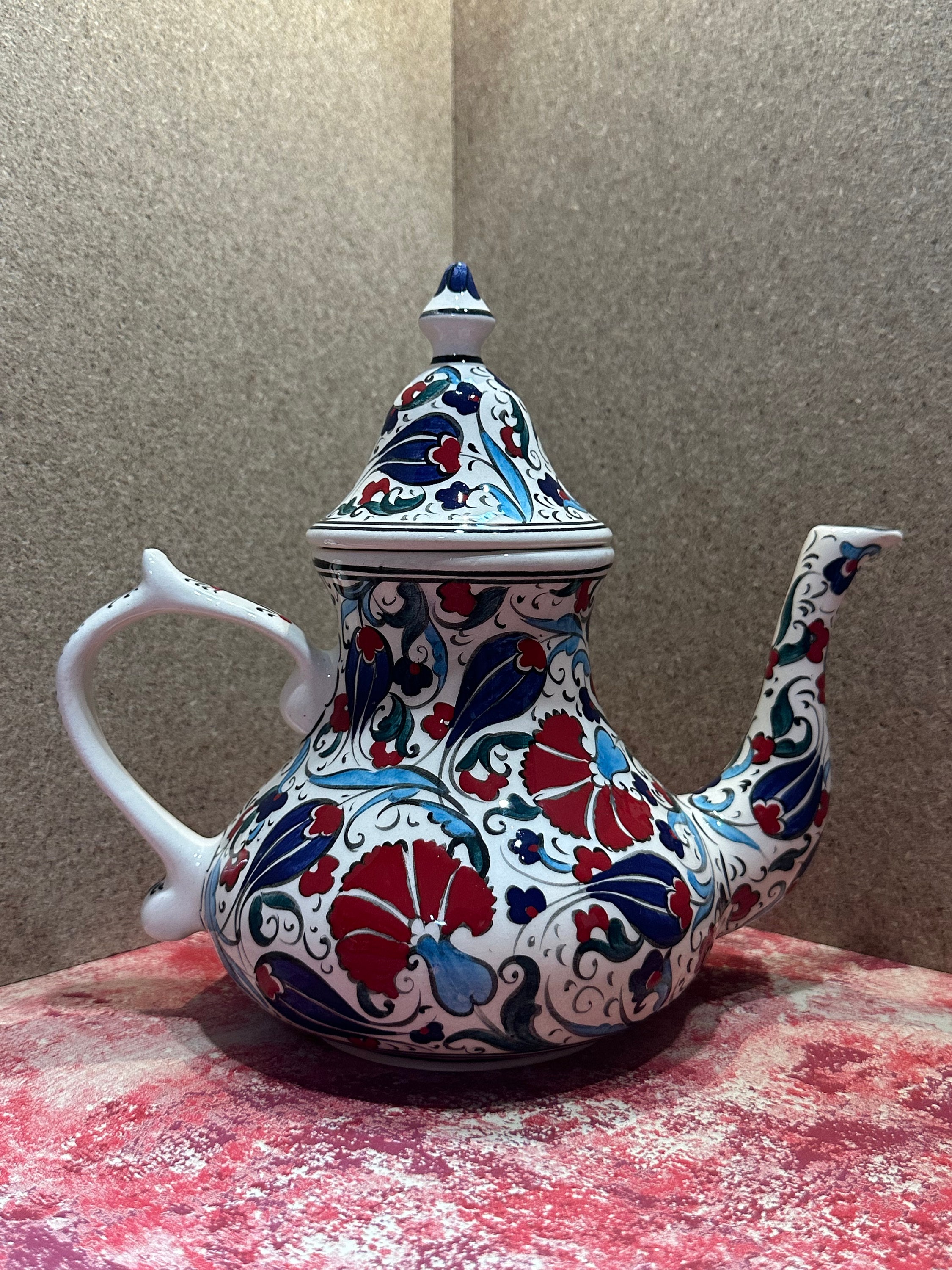This photograph showcases a large, ornately decorated teapot, possibly on display in a museum. The teapot stands out with its white base and intricate designs featuring mushroom-like motifs where the trunks are light blue, and the branches and flowers are dark red. Complementing these motifs are scroll designs in shades of turquoise and navy blue. The teapot is adorned with a high, removable lid topped with a blue knob, and it sports a substantial handle on the left and an elegantly curved spout on the right.

The teapot is placed on a multicolored, textured surface that ranges from burgundy red to lighter reds, pinks, and whites, giving the impression of a neatly executed paint splatter. The background features walls that appear to be a speckled pattern of grays, evoking a stone-like or cork-like appearance. The setting contributes to the overall display, enhancing the handcrafted aesthetic of the teapot with its nature-inspired design.